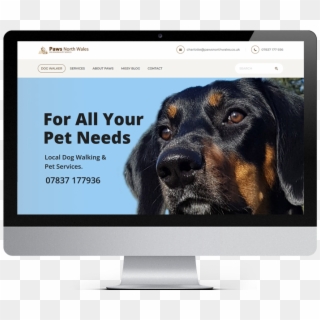This image depicts a computer screen displaying a website with a white banner at the top. The website is titled "PAWS," spelled out in capital letters, P-A-W-S. Beneath this banner, there are various navigation tabs, though they are faint and somewhat unreadable. A partially obscured web address and a contact number are present, accompanied by a circular phone icon.

The main backdrop of the page is light blue. Dominating the right half of the screen is a large image of a black dog, prominently featured and occupying more than half of the on-screen space. Adjacent to the dog's image, text reads, "For All Your Pet Needs," followed by "Local Dog Walking and Pet Services." At the bottom, a phone number is provided, formatted as 07837 177936.